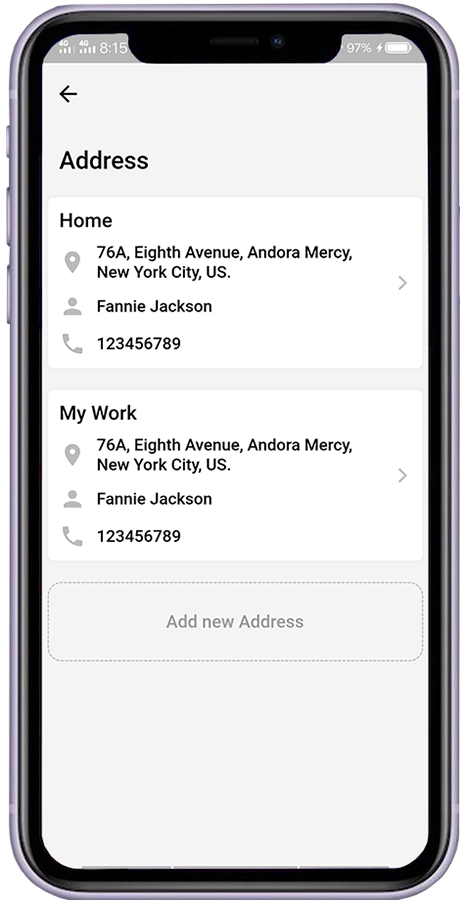The image features a gray-colored smartphone with a black outline, set against a gray background. At the very top of the screen, the status bar displays the time "8:15" and the battery at "97%". Below the status bar, there is a light gray box containing a left arrow icon and the word "Address".

Underneath this, there is a white box labeled "Home," which contains the address "76A 8th Avenue, Andorra, Mercy, New York City, US." It also lists a name, "Fannie Jackson," and a placeholder phone number, "1 2 3 4 5 6 7 8 9," accompanied by a right arrow icon.

A light gray division separates this from another white box, labeled "My Work," which repeats the same address, "76A 8th Avenue, Andorra, Mercy, New York City, US," name, "Fannie Jackson," and placeholder phone number, "1 2 3 4 5 6 7 8 9."

At the bottom, another light gray area includes a small box with the text "Add new address" in light gray print.